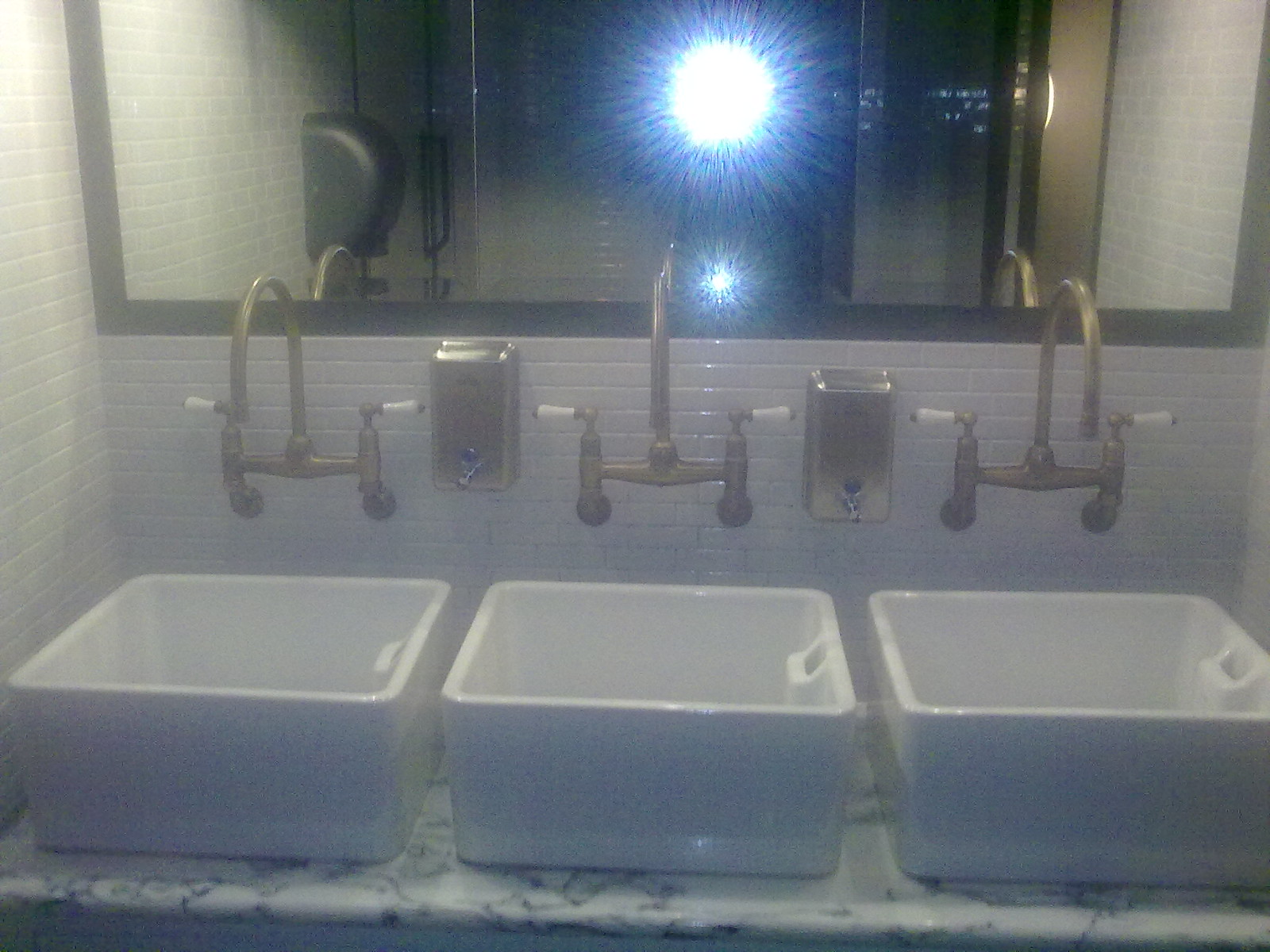This photo showcases a modern public bathroom with three large, square white porcelain sinks, each about eight inches tall, lined up in a row on a white and gray marble countertop. The sinks are complemented by ornate, upside-down U-shaped brass faucets with white handles for hot and cold water. Situated between the sinks, there are two silver metallic soap dispensers, with one positioned slightly higher than the other. Above the sinks, a gray-rimmed mirror reflects the bright flash from the camera, revealing a gray, rounded paper towel dispenser on the left wall. The surrounding walls are adorned with small, off-white tiles. Overall, the scene captures a meticulously detailed and elegant bathroom setup.